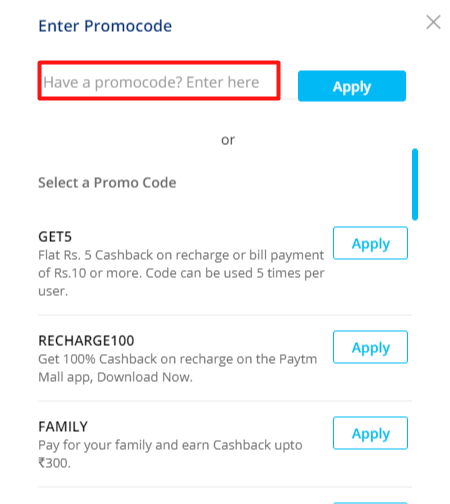**Detailed Caption:**

The image showcases a mobile phone screenshot of a checkout page from a website, displayed in portrait orientation against a white background without any defined borders. At the top, there is a blue header with the text "Enter Promo Code," complemented by an 'X' icon in the upper right corner for closing the promo code section. Below the header, a prominent, long red rectangular box features the text "Have a promo code? Enter here."

Directly beneath the red box, there is a long blue rectangular button with white text that reads "Apply." Centered underneath this button is the word "or" in grey font. Below the "or," another instruction appears in grey text, stating "Select Promo Code," paired with a light blue toggle arrow on the right side of the page, possibly indicating a dropdown menu.

The page provides three promotional options, each separated by a thin grey border. The first promotional offer reads: "Get flat Rs. 5 cashback on recharge or bill payment of Rs. 10 or more. Code can be used five times per user," accompanied by a blue rectangular "Apply" button.

The second offer says: "Recharge 100 and get Rs. 100 cashback on recharge on the Paytm Mall app. Download now," also featuring the same blue "Apply" button.

The third promotional offer promotes: "Family Pay: Pay for your family and earn cashback up to Rs. 300," followed by another blue "Apply" button.